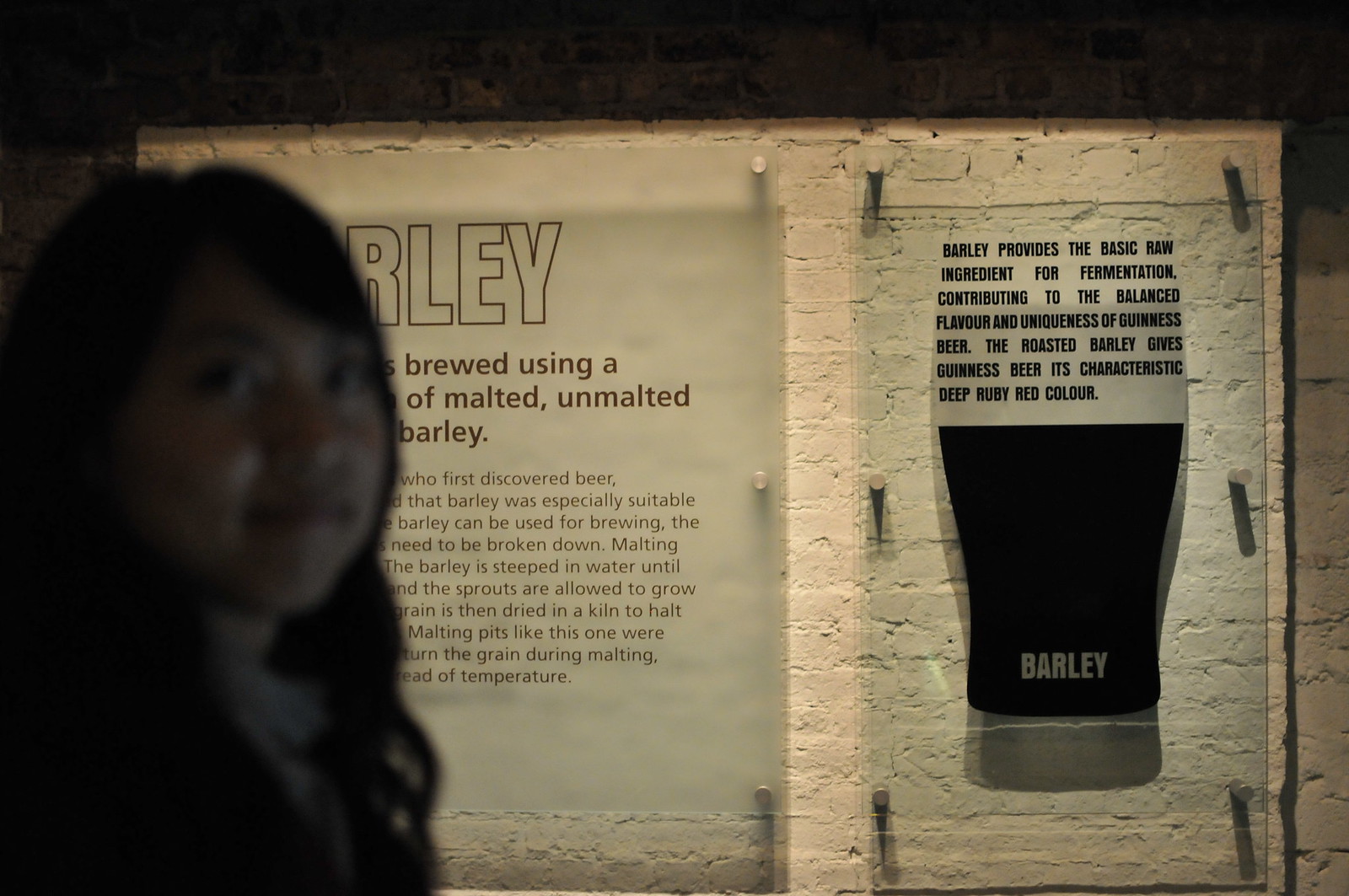In a dimly lit room, a concrete wall serves as the backdrop for an informative display about barley's significance in brewing Guinness beer. The focal point of the image is a large depiction of a beer glass, prominently showing the signature deep ruby red color of Guinness, topped with a white frothy head. The text on the wall reads, "Barley provides the basic raw ingredient for fermentation, contributing to the balanced flavor and uniqueness of Guinness beer. The roasted barley gives Guinness beer its characteristic deep ruby red color." 

A young woman with long dark hair, dressed in a light-colored shirt, stands to the left of the display. She smiles while looking at the camera, partially obscuring a portion of the text that begins with "barley." The background is predominantly black, highlighting the white and beige tones of the wall and text, making the informative content stand out. The ambiance and the detailed display suggest that this photo could have been taken at the Guinness Brewery or a related museum exhibit.